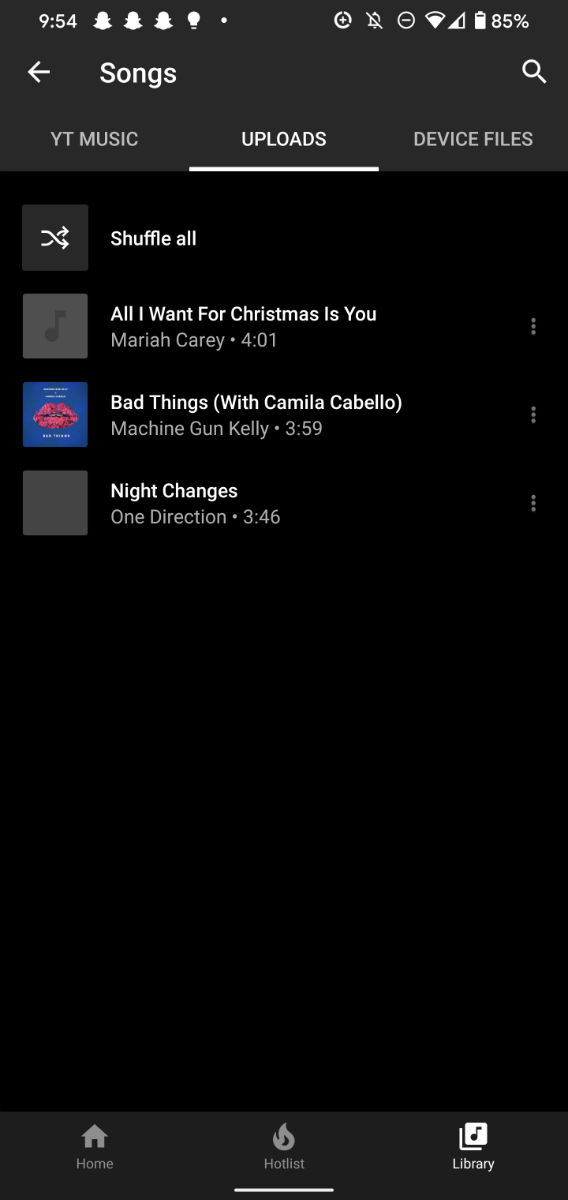This is a detailed screenshot taken from a mobile device. The screen displays the YouTube Music app interface at 9:54 PM with 85% battery life remaining. The top part of the screen features a search bar, all set against a black background with white text. The interface is in "Songs" mode, indicated by a left-pointing arrow. The sidebar shows navigation options including "YT Music," "Uploads," and "Device Files."

A shuffle button is also present. The first song listed is "All I Want for Christmas is You" by Mariah Carey, followed by "Bad Things" featuring Camila Cabello and Machine Gun Kelly, and lastly, "Night Changes" by One Direction. At the bottom of the screen are navigation buttons for "Home," "Hotlist," and "Library" with a musical note icon.